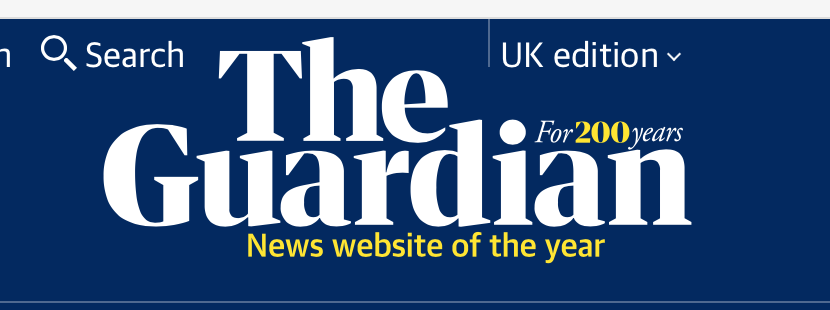The image is a screenshot of a section of The Guardian's website, primarily showcasing its header. The background is a navy blue rectangle, suggesting it is part of the website's top section. 

Prominently displayed in the header is The Guardian's iconic logo: "The Guardian" is written in a clean, white font. "The" appears above "Guardian," positioned between the letters 'U' and 'A.' Beneath the main logo, in yellow font, it proudly states "News Website of the Year." Additionally, above the 'A' and 'N' in "Guardian," the number "200" is highlighted in yellow, celebrating "200 years" of the publication, with "for" and "years" written in italicized white font.

To the upper left, also in white but non-bold font, it says "search" beside a search icon. Above the main header in white font, the text "UK edition" is visible, accompanied by a downward arrow indicating a drop-down menu. The overall design is sleek, showcasing significant accolades and features succinctly.